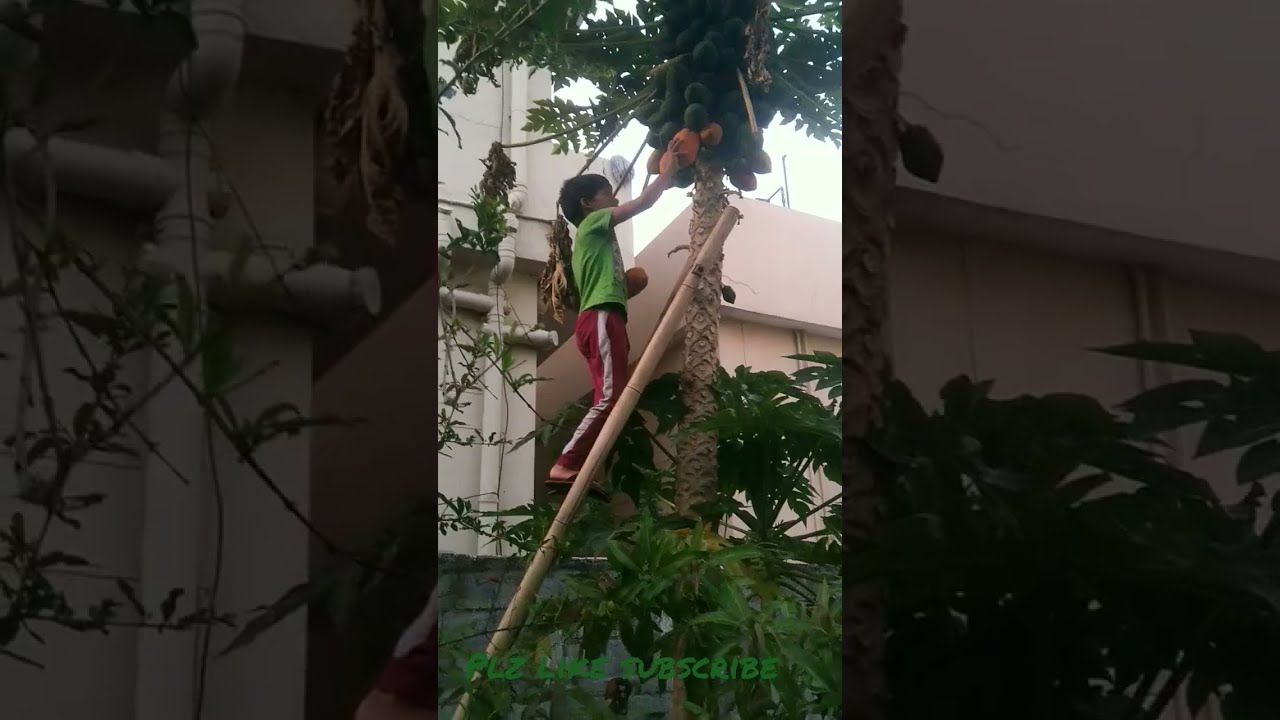In the image, a young boy, approximately 9 or 10 years old, is depicted climbing a wooden ladder to pick fruit from a tree. He has short black hair and is dressed in a green shirt paired with red track pants featuring a white stripe down the sides, and sandals. The boy, using his right hand, is holding an orange fruit while reaching for another amidst a mix of ripe orange and unripe green fruits. The fruit tree has a thin, light brown trunk, resembling a tropical tree or a thin palm, and its foliage spreads densely to the right and sparsely to the left. The scene is set during the daytime under the bright sun, revealing a two-story white building and a single-story light pink building in the background. Additionally, more greenery and white piping are visible, along with text at the bottom of the image that reads, "Please like and subscribe" in green.